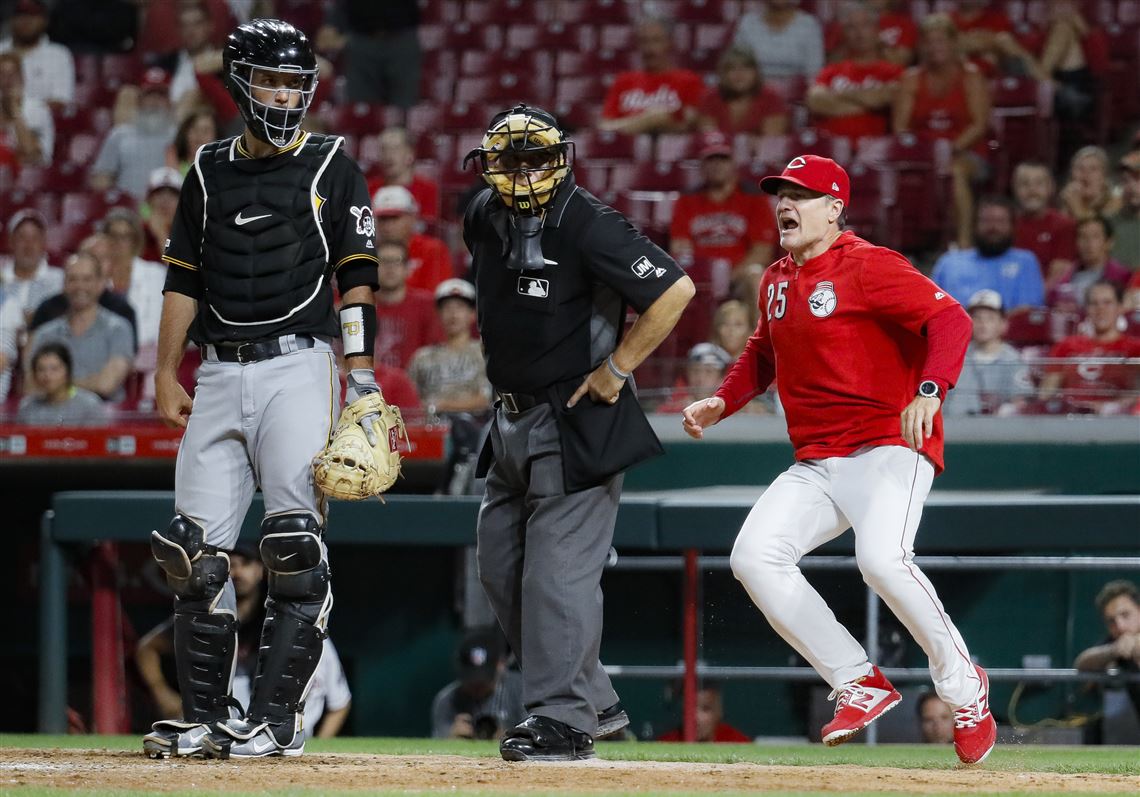In this detailed depiction of a Major League Baseball scene, we observe an intense moment at the forefront. At the heart of the action stands an umpire, distinguished by his black shirt, helmet with a yellow face guard, black pouch hanging from his belt, gray slacks, and black shoes. To his left, the catcher, donned in a black uniform, gray pants, and a black helmet, is fully geared with shin protectors and a chest pad featuring a Nike emblem. Displaying raw emotion and fervor to the right of the umpire is the Cincinnati Reds manager, believed to be Pete Rose. He wears a bright red cap, a red zip-up sweatshirt with the number 25 and the team's mascot on the left side, gray pants, and red New Balance shoes. His mouth wide open, he's visibly agitated, likely disputing a controversial call with the umpire. This compelling scene unfolds against a backdrop of an almost empty stadium, with scattered fans, predominantly clad in red, cheering from the front rows. The vibrant green grass of the outfield, the dirt infield, and the dugout with observing players encapsulate the vibrant atmosphere of the game.